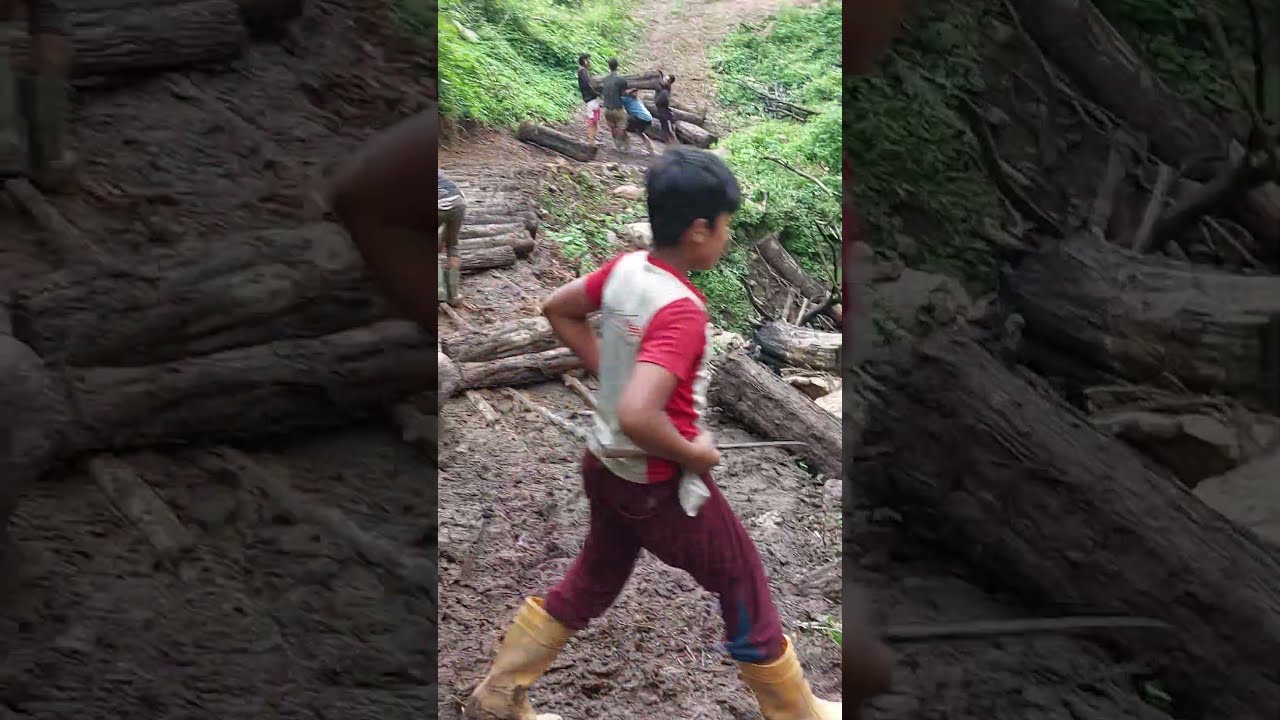The image captures a scene in a forested area with a central trail lined by logs and shrubbery on either side. The foreground focuses on an Indian boy with dark hair, who is performing a forward lunge, his right leg stretching towards the three o'clock direction. He wears a white short-sleeved shirt with red sleeves, maroon pants, and high yellow boots. The boy's hands rest on his hips as he stands on a grounding of wood chips or dirt, surrounded by logs. In the background, a few individuals, possibly workers, are visible lifting or carrying logs further down the trail. The side edges of the image are blurred or dimmed, emphasizing the central activity. The overall setting is a wooded environment with a color palette featuring brown, yellow, maroon, red, white, green, and blue hues, and the style suggests it may have been captured as a screenshot from a mobile device.